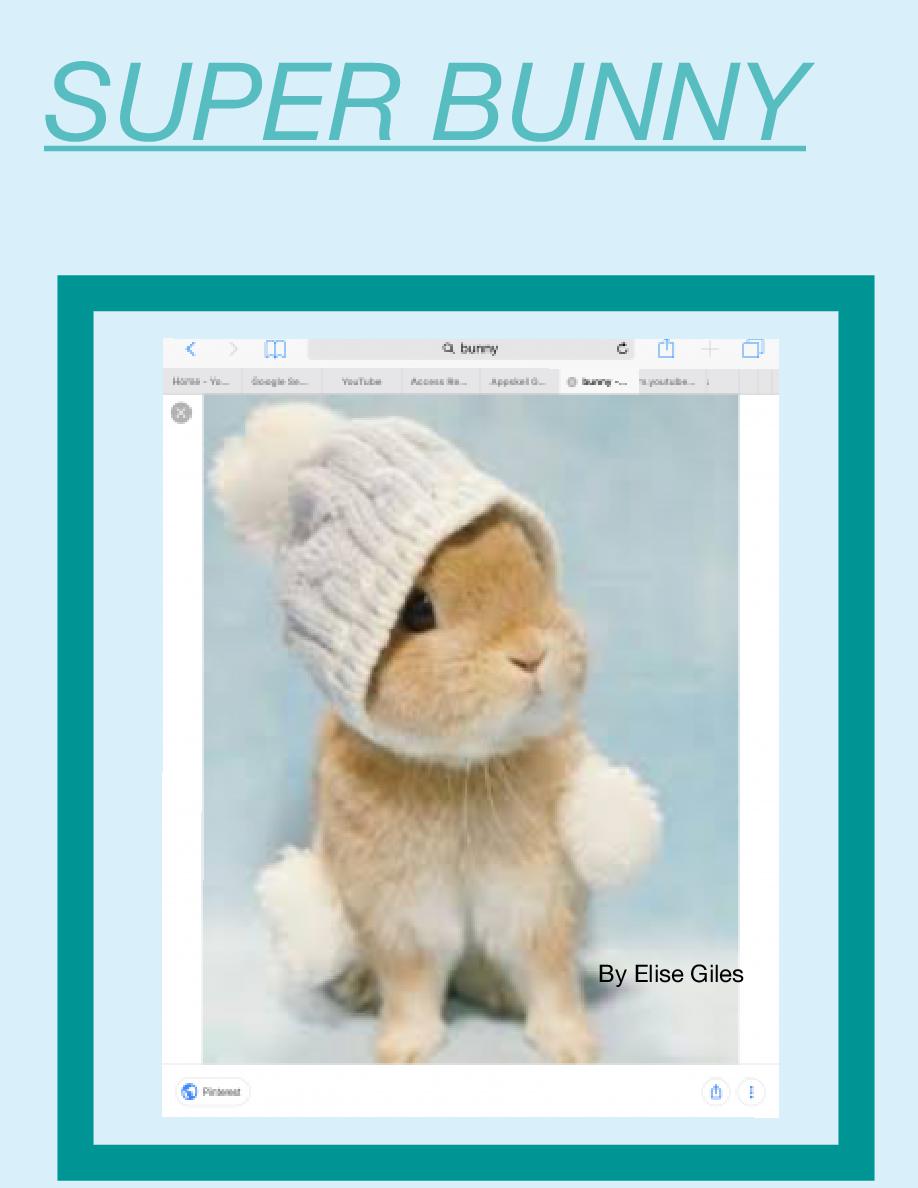The image depicts a webpage displayed on an iPad screen. The primary focus is a large, light blue rectangle filling the background. At the top of this rectangle, the title "SUPER BUNNY" is prominently written in capitalized aqua font and is underlined. Surrounding the main content is an aqua border, which is quite thick and square-shaped. Inside this, there is an even thicker light blue border.

At the top of the webpage, navigation elements are visible. The left side features a blue back arrow button, while the right side shows a light gray forward arrow indicating it is disabled. Next to these, toward the right, is a bookmarks icon resembling a blue-outlined book. The search bar, though slightly blurry, contains the text "bunny BUNNY". Following the search bar are various icons: a refresh symbol, a blue share symbol (a rectangle with an upward-pointing arrow), a disabled cross button, and a Windows button.

Several tabs are open on the browser; however, only two are legible: one labeled "YouTube" and another with the word "access."

Central to the webpage is an image of a bunny wearing a stocking hat with a pom-pom at the top and two more at the ends of strings hanging from the hat. The bunny is gazing to the side. Below the image, towards the right side, the text "by Elise Elise Giles" is displayed. On the bottom left, there is a rounded rectangular button labeled "Pinterest" alongside a globe icon.